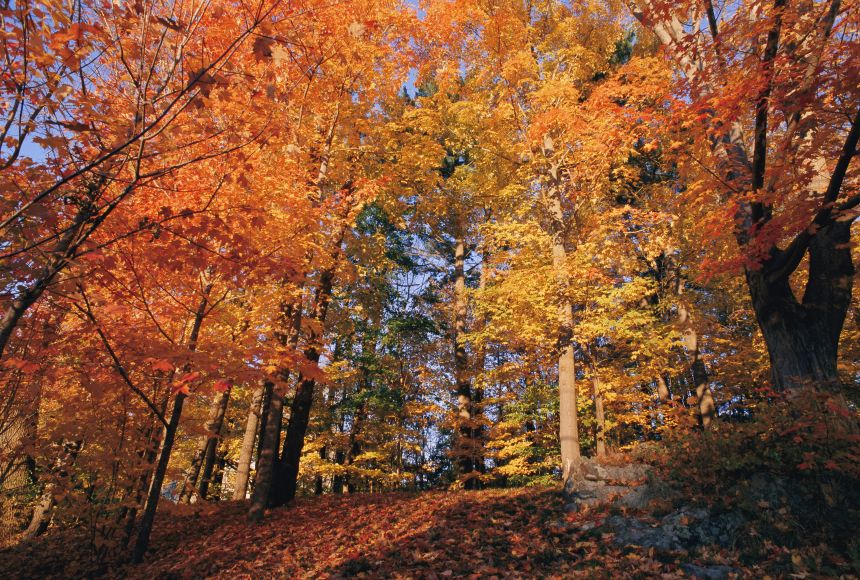The photograph captures a serene autumnal scene in a forest, where the vibrant transition of leaves marks the fall season. Dominating the image are deciduous trees with trunks of varying sizes and a mix of yellow, orange, brown, and red leaves. Some trees, especially those towards the back, retain more green leaves, highlighting the gradual shift of the season. The trees in the middle showcase a stunning array of fall colors, with the tree on the left having a mix of orange and light brown leaves, and the one in the middle featuring orange and yellow leaves. Fallen leaves blanket the forest floor, matching the canopy's hues. Amidst the foliage, a green bush stands in the foreground, and a gray rock is visible to the right. The sky, a clear light blue, peeks through the trees, with no clouds in sight. Sunlight filters through the branches, casting a warm glow on the picturesque scene, embodying the essence of a peaceful autumn day in the forest.